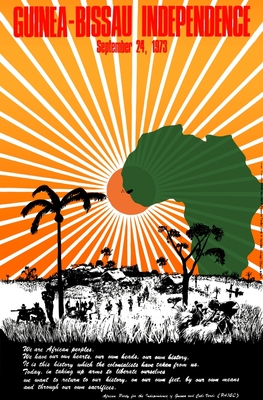The image is a detailed poster commemorating Guinea-Bissau's Independence on September 24th, 1973. At the top, bold red text announces "GUINEA-BISSAU INDEPENDENCE." Directly below the title, the significant date is displayed in matching red font. Dominating the center of the poster is a vibrant orange sun, with white rays radiating from it, symbolizing the dawn of a new era. On the right side of the image, a green shape hints at a map of Africa, anchoring the visual context. The left corner features a palm tree with a visible coconut, adding a tropical touch to the scene. Silhouetted human figures occupy the lower part of the poster, though their identities and details are indiscernible. Scattered rooftops of small houses are seen in black and white, providing a subtle background contrast. The bottom of the poster contains small white text on a black strip, but it remains illegible due to its size and blurriness. The overall color palette includes shades of orange, green, black, red, and white, reflecting the significance and vibrancy of the occasion.